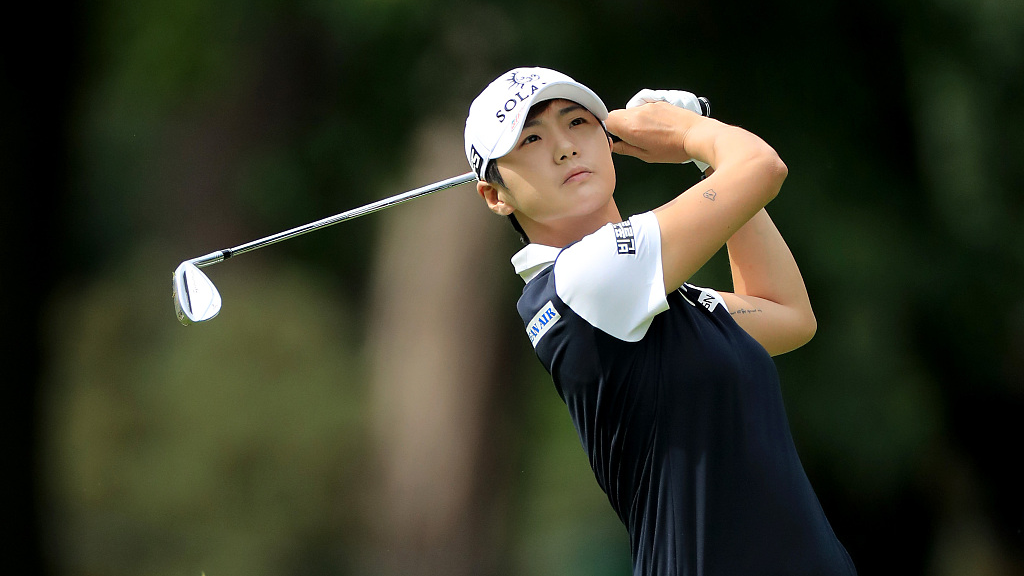This detailed image captures a golfer, potentially identified as Yee-Lee-Me-No at the Portland Classic golf tournament. The golfer is Asian, likely Chinese, and is sporting a distinctive white hat with "SOLA" partially visible on it. Dressed in a blue, short-sleeved shirt with white collar and sleeves, the back of the shirt displays the word "AIR", possibly to promote clean air. The golfer is holding a silver golf club, with both arms bent at the elbows and raised up in the air in a follow-through position, indicating a recently completed swing. Visible tattoos include a small one on the outside of the right arm and another on the inside of the left arm. The background is out of focus, but a tree can be seen, emphasizing the outdoor setting of a golf course.